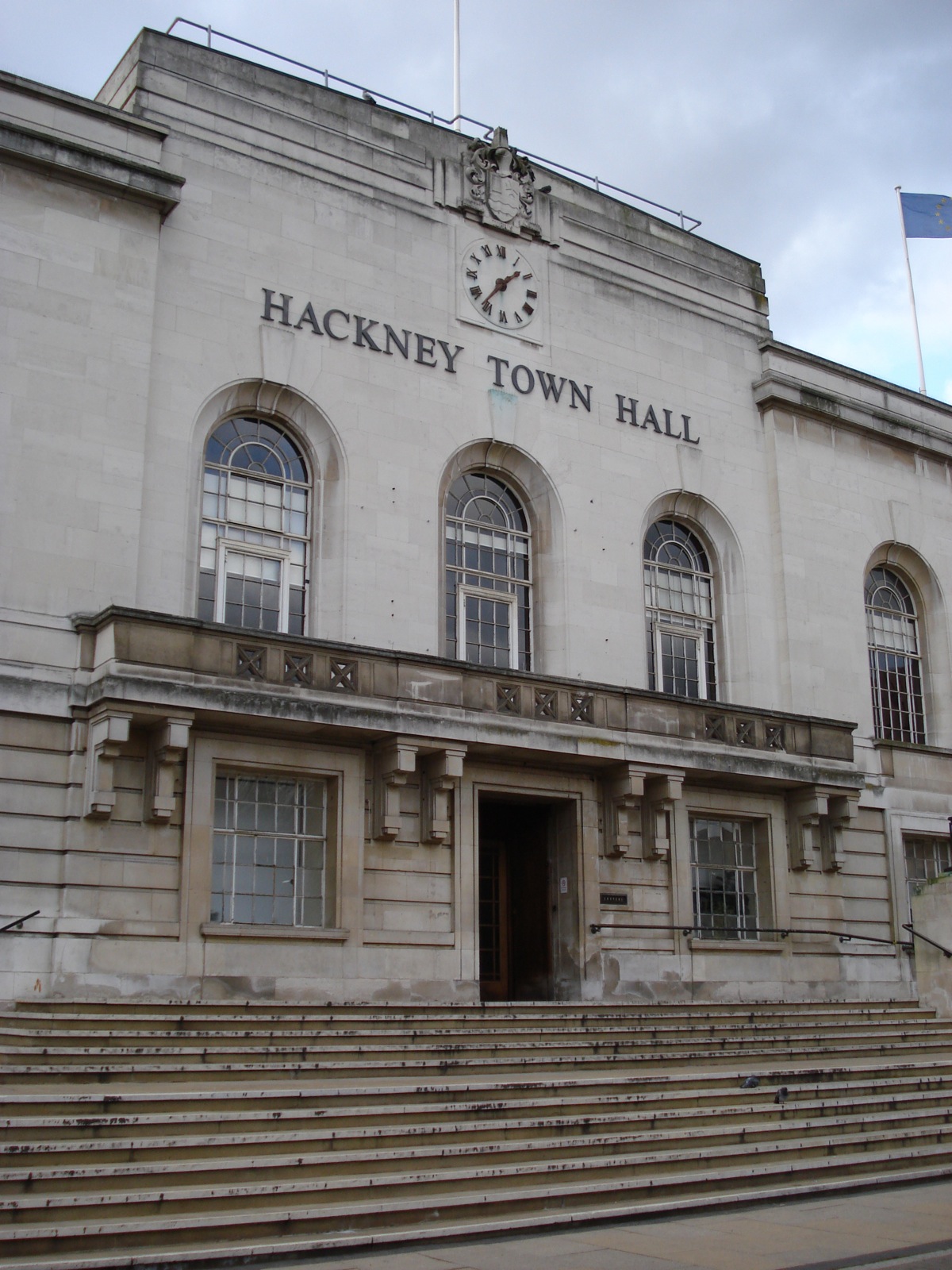This photo depicts the stately Hackney Town Hall, an aged and weathered building constructed from large stone and concrete. Centered above the main entrance, three large arched windows add a grandiose touch, accompanied by an elegant balcony perched below them. The balcony sits right above the main door, which is flanked by two glass windows. To reach the entrance from the street, visitors must ascend two flights of steps, each comprising at least five steps. A notable feature is the clock mounted in the wall above the "Hackney Town Hall" sign, adding a historical charm. Additionally, a blue flag is visible flying on the right-hand rooftop, hinting at the building's civic significance. The top portion of the building appears to be made from poured concrete, in contrast to the robust stone masonry at the bottom, emphasizing its durable construction. The photo is a front view shot, taken from ground level, capturing the full, imposing facade of this historic town hall.